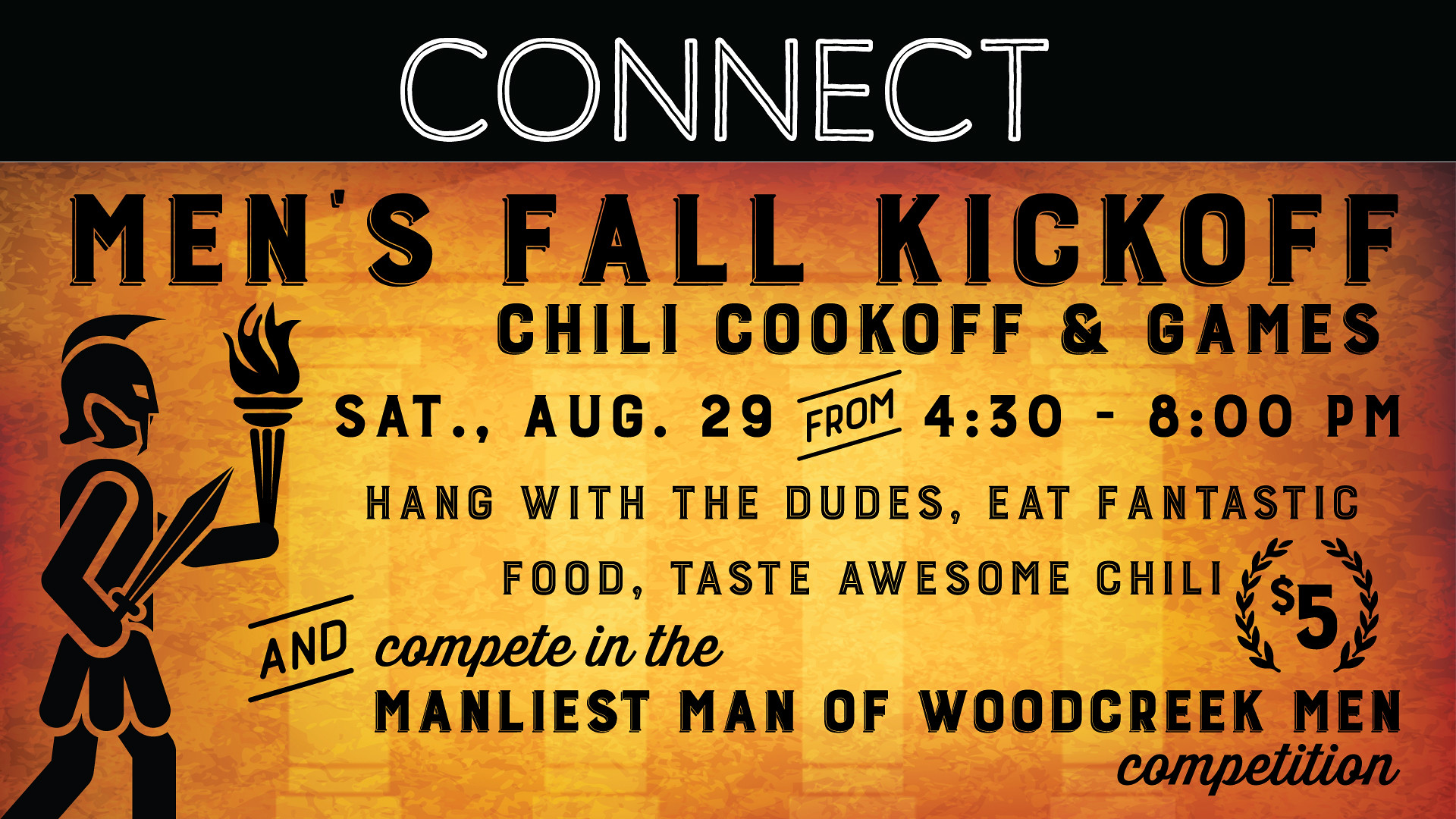The promotional image for the Men's Fall Kickoff event prominently features the word "Connect" in bold white text on a black banner at the top. Below, the background shifts to a golden hue adorned with Greco-Roman pillars. The primary event details are displayed in uppercase black text, announcing: "Men's Fall Kickoff Chili Cook-Off and Games." The date and time, "Saturday, August 29th from 4:30 to 8 PM," are noted underneath. The event invites participants to "Hang with the dudes, eat fantastic food, taste awesome chili," with an entry fee presented as "$5" within a laurel wreath. Additionally, attendees can "compete in the Manliest Man of Wood Creek Men's Competition." Complementing the text is a rudimentary yet detailed drawing of an ancient soldier in a steel uniform, wielding a sword in his right hand and an Olympic torch in his left.